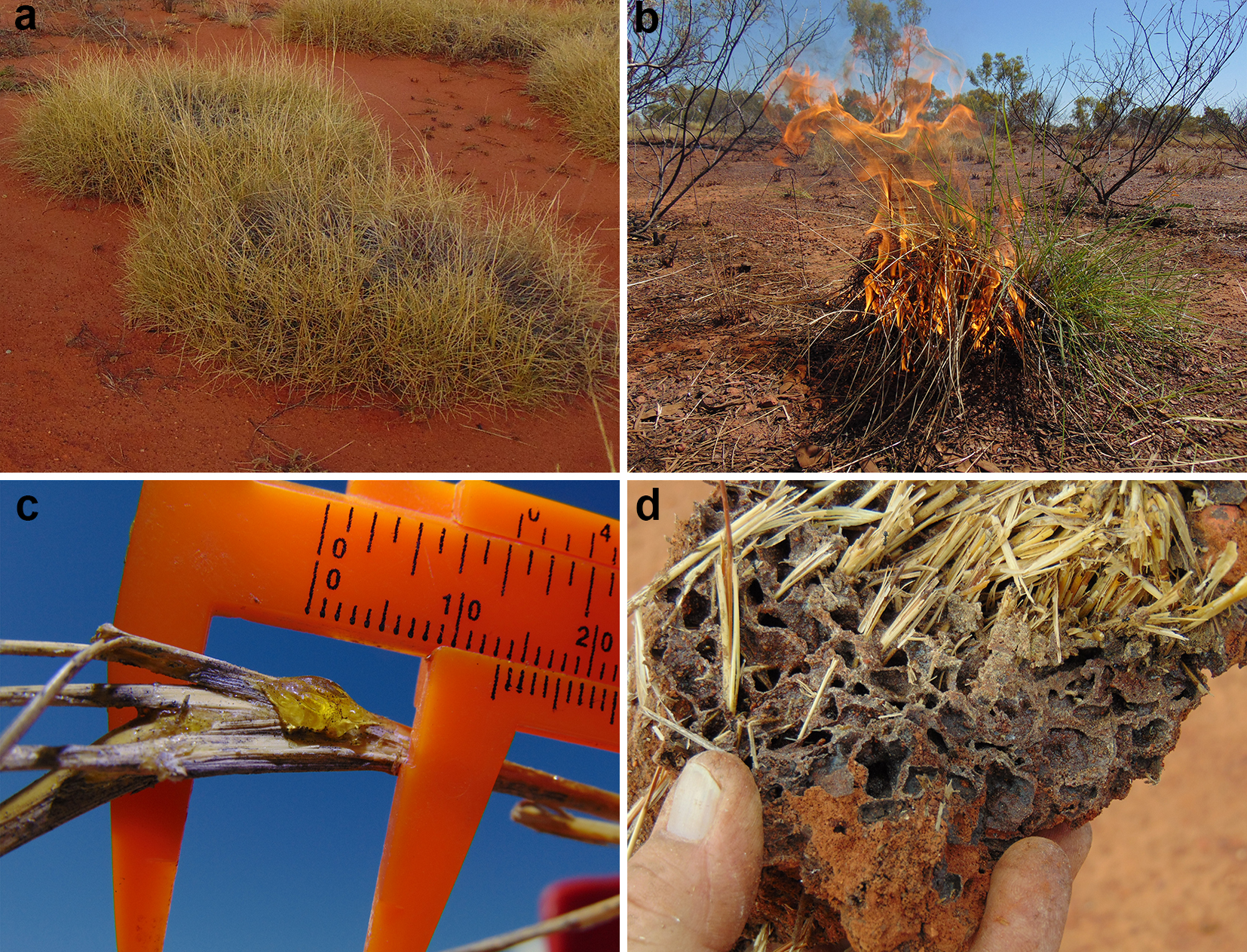The series comprises four nature-related photographs, labeled A, B, C, and D. In the top left (A), a desert-like terrain with patches of yellow and brown dry grass is prominent against a clay-colored ground. To its right (B), a controlled fire ignites dry twigs, with orange flames rising amidst a dry landscape dotted with some greenery and clear skies. Below on the left (C), an orange caliper measures a stick, which appears to have a bug or cocoon on it, with visible black measurement markings. Finally, in the bottom right (D), a hand holds what seems to be a bee or wasp nest, partially embedded in dry grass and brown clay, suggesting it was extracted from the ground.